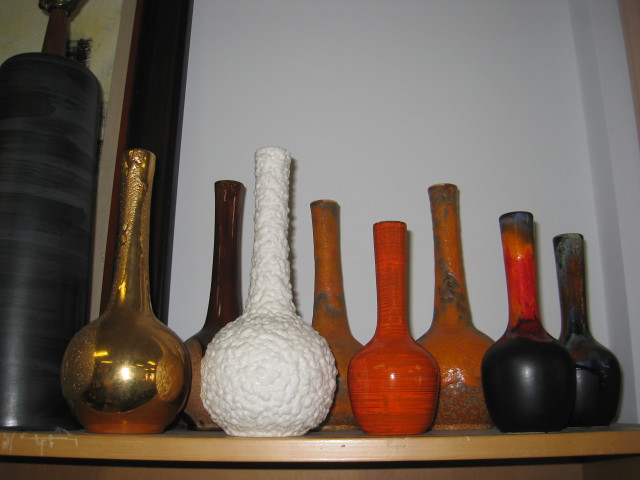The photograph showcases a collection of eight intricately designed vases arranged in two rows of four on a brown wooden shelf, set against a featureless white wall. To the left, there's a large black vase with gray streaks and a brown top, standing next to a shiny bronze vase that transitions from a spherical bottom to a cylindrical neck. Adjacent to these is a white ceramic vase with a rough texture, partially obscuring another vase that blends light and dark brown hues. 

Continuing rightward, an orange vase with dark gray streaks stands prominently. Beside it is a red vase with maroon streaks, resembling a bowling pin in shape. Flanking these is a black vase with a red body, streaked with orange, greenish-yellow, light blue, and dark blue hues towards the top. The final piece in the lineup is a black vase adorned with patterns of orange, blue, green, and gray. All the vases feature round bottoms and slender, elongated necks, creating a cohesive yet varied aesthetic on the wooden shelf.